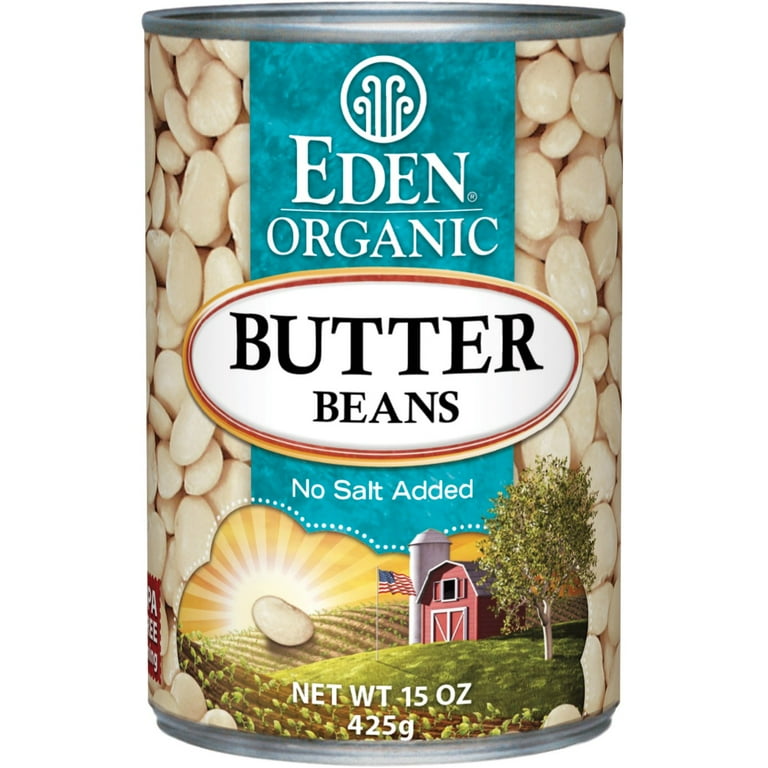This image features a 15-ounce (425 grams) can of Eden Organic Butter Beans, with no salt added. The can prominently displays the product name in a large, white oval with black lettering and outlines. Above the oval, "Eden Organic" is printed in dark blue. The can's background is covered with images of whitish-beige butter beans. Near the bottom of the can, there's a detailed and picturesque graphic of a farm scene. The farm includes a red barn with a white silo to its left, a tree with white bark (possibly a birch tree) to its right, and lush green crops growing across the field. An American flag is proudly displayed on a flagpole in front of the barn, and the whole scene is set against a sunlit backdrop with green grass.